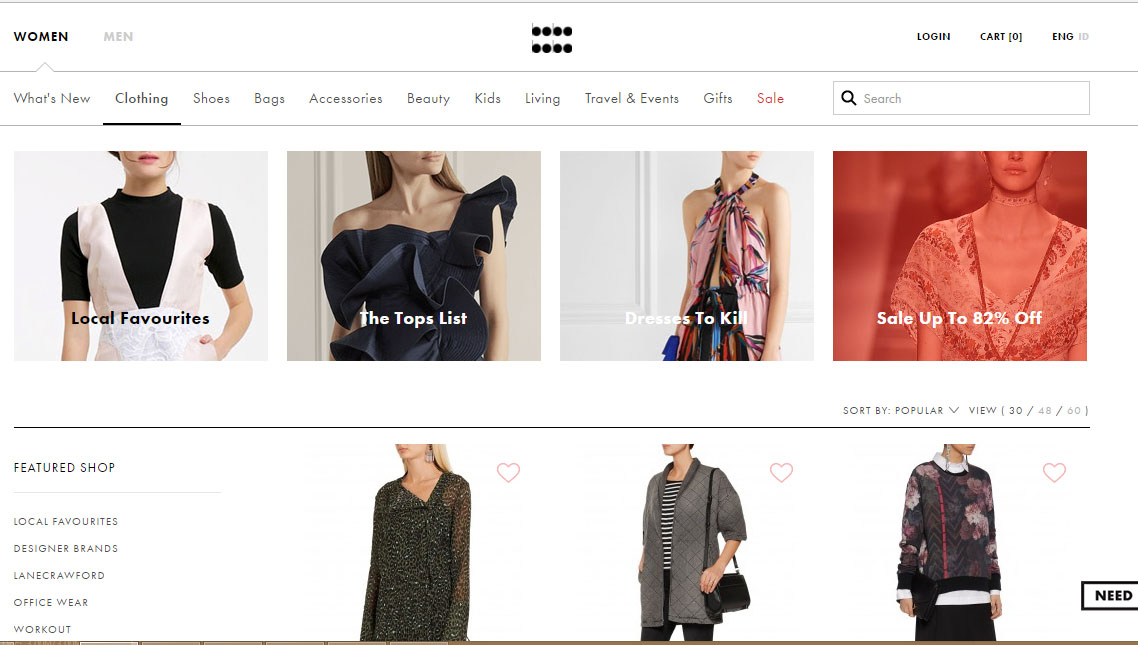A white rectangular header spans across the top of the image. The header features a light gray line running horizontally from edge to edge. Directly beneath this line, the words "Woman" and "Men" are displayed, with "Woman" in black text and "Men" in gray. Aligned to the right side, the text "Login," "Cart (0)," and "ENG HD" is present. A second gray line follows below, separating this section from the navigation menu.

The navigation menu reads: "What's New," "Clothing," "Shoes," "Bags," "Accessories," "Beauty," "Kids," "Living," "Traveling," "Events," "Gifts," and "Sale," with the word "Sale" highlighted in red, while the rest are in black. Alongside this menu is a search button.

Beneath the navigation menu are four square images, each representing different categories. The first is labeled "Local Favorites" and depicts a woman in a black short-sleeve shirt layered under a sleeveless dress. The second square is titled "Top List" showcasing a woman in a chic one-shoulder dress, with one shoulder covered and the other bare. The third square, "Dresses to Kill," presents a vibrant pink dress adorned with black, red, blue, and gold hues, wrapping elegantly around the model's neck. The fourth square, marked "Up to 80% Off," is shaded red and features a floral V-neck dress in the background.

Below these squares are three additional photos of women modeling different outfits. The first image shows a woman in a black sparkly dress. The second depicts a woman in a gray jacket over a black and white striped shirt, accessorized with a black purse slung over her shoulder. The third image features a woman wearing a white long-sleeve shirt beneath a black sweater decorated with white, gray, and red flowers.

A bold black line separates this section from whatever content lies below.